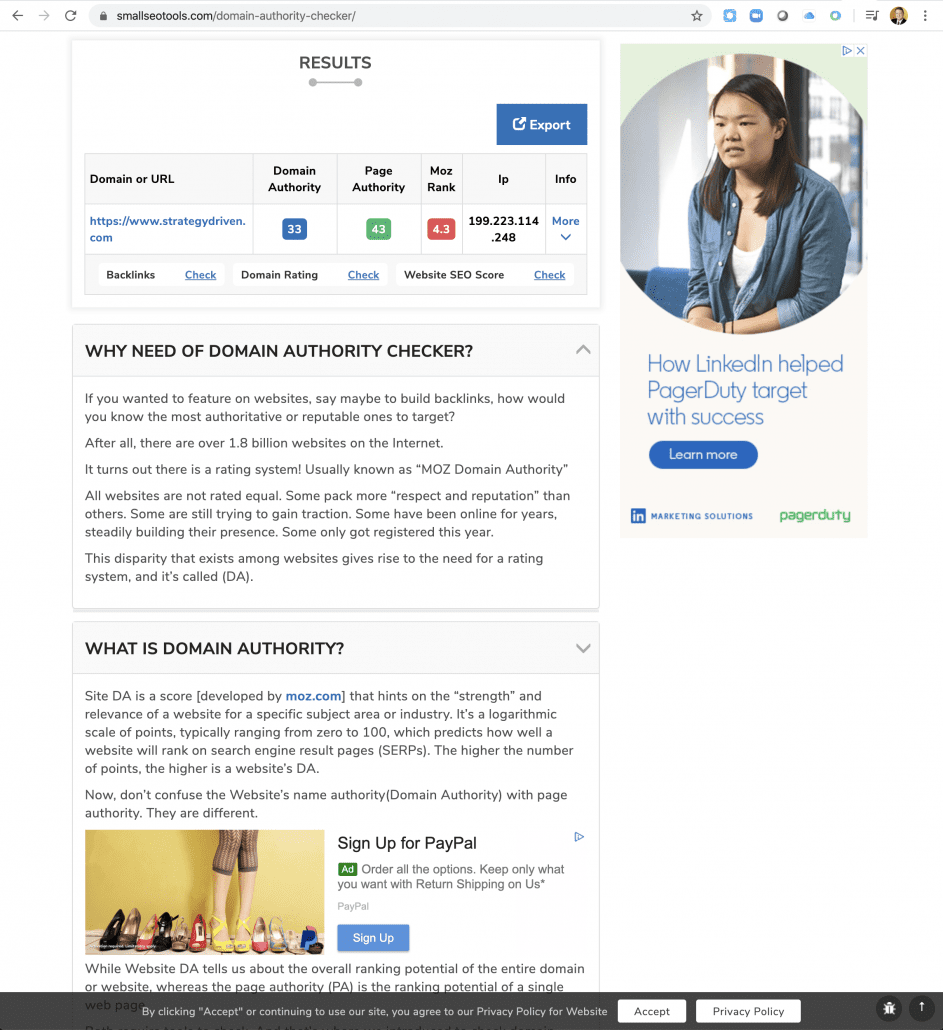The image showcases a web browser displaying the "Domain Authority Checker" tool on SmallSEOTools.com. At the top of the browser, there is a navigation bar with a white background. It contains a black arrow pointing left, a gray arrow pointing right, and a black circular arrow symbolizing refresh.

In the address bar, a gray lock icon is present, followed by the URL "smallseotools.com/domain-authority-checker/". There is a star icon with a white center and gray border next to the URL.

Below the navigation bar, the screen is mostly white with a section titled "Results" in gray, underlined by a gray line segment. On the right side, a blue rectangle with white text reads "Export."

Under the "Results" section, the following columns are displayed:
- "Domain or URL" in black
- "Domain Authority" in black
- "Page Authority" in black
- "MOZ Rank" in black
- "IP" in black
- "Info" in black

The results show the following data:
- In blue, "https://www.strategydriven.com"
- In white, "33"
- In white, "43"
- In white, "4.3"
- In black, "199.223.114.1"
- In blue, "More"

At the bottom of the results, there are several options in black and blue text:
- "Black Links" in black with "Check" in blue next to it
- "Domain Rating" in black with "Check" in blue next to it
- "Website SEO Score" in black with "Check" in blue next to it